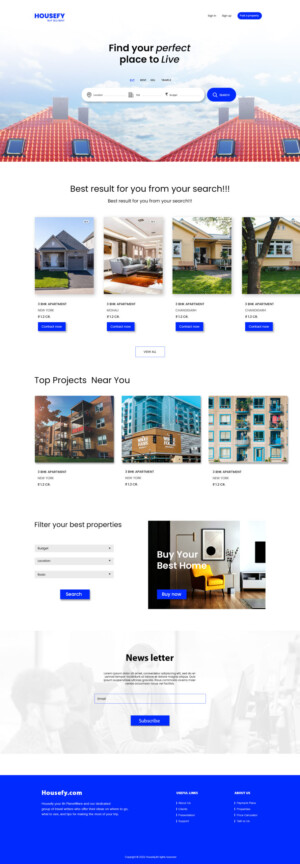This screenshot is from the mobile version of the Houseify website. The webpage, presented in a vertical format indicative of a smartphone display, offers a detailed and user-friendly interface for searching homes to buy or rent. At the top left corner, the distinctive blue Houseify logo and name are prominently displayed. On the top right, users can access links to log in, sign up, or find a property.

Below the header in black text, the site encourages users with the phrase "Find your perfect place to live." Directly beneath this, there's a white search dialog box enabling users to input a location, specify the type of property, and set a price range. This search function is accompanied by a blue button labeled "Search," iconized with a magnifying glass.

The page's background is aesthetically pleasing, featuring images of two homes with red roofs set against a serene blue sky with white clouds, reinforcing the site’s real estate theme. Below the search section, there's text that reads "Best results for you from your search," indicating the property listings section.

Here, four different properties are displayed, each accompanied by pertinent details such as the property name, location, and rental price. A blue button is present on each listing, presumably leading to more detailed information about the respective property, although the text on this button is not clearly legible.

Further down the page, a row of three images titled "Top projects near you" showcases large apartment buildings available for rent. The user can explore these options as well.

At the bottom part of the page, additional functionalities are provided, including options to filter properties, buy the best home, and sign up for a newsletter. The footer in a blue box offers links to essential information about Houseify, such as company details, career opportunities, privacy policies, and more.

This comprehensive and visually appealing layout ensures users can easily navigate and find relevant property information.